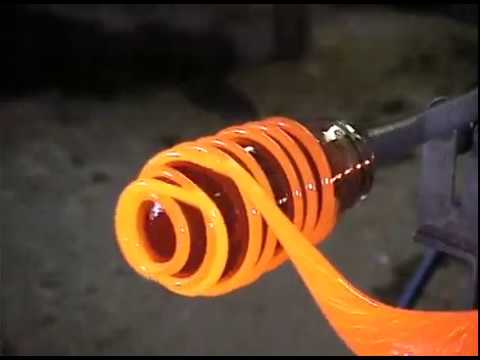The image depicts a scene from a glass-making process, likely set in a factory environment with a gray ground surface. A dark, iron-colored metal apparatus, resembling a honey wand, extends from the right-hand side. At the end of this rod, molten glass in a radiant spectrum of bright orange to yellow is being meticulously twirled into a spiral pattern. The glowing material has a wet, melted appearance and is wrapped around the cylinder of the rod, forming intricate circular strands. In the background, shadows can be observed, hinting at an outdoor light source or open space within the factory setting.